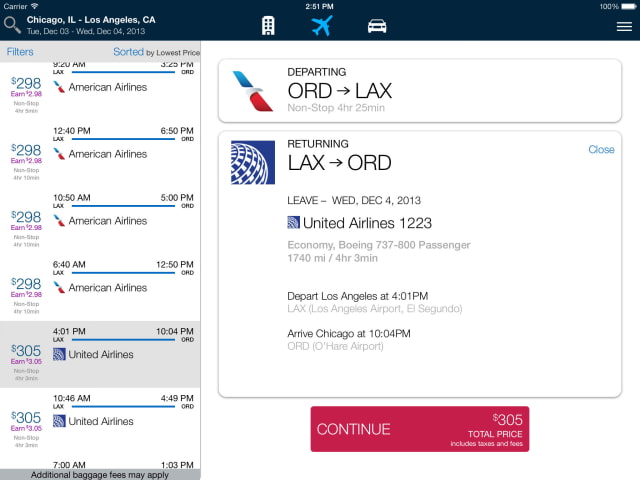A detailed and cleaned-up caption for the image could be:

---

The image features a flight itinerary with a white background. It includes a magnifying glass icon showing a 100% battery status. The itinerary details a flight from Chicago, IL (ORD) to Los Angeles, CA (LAX) scheduled for a 4-hour and 25-minute non-stop journey. The departure from ORD is marked with a right arrow, indicating a direct flight to LAX. It departs on Wednesday, December 4, 2013, at 2:51 PM from Chicago and arrives in Los Angeles at 4:41 PM. 

The return flight from Los Angeles to Chicago departs LAX at 10:04 PM and arrives at ORD, highlighted with a right arrow. The itinerary mentions the use of a United Airlines Boeing 737-800, flying a total distance of 1,740 miles. The fare is listed in Economy class as $305, marked with a red rectangle containing the word "Continue." The blue-colored parts of the image include the airplane and car icons, alongside the highlighted "Closed" status and departure information.

---

This caption precisely describes the elements in the image, emphasizing key details about the itinerary and visual components.